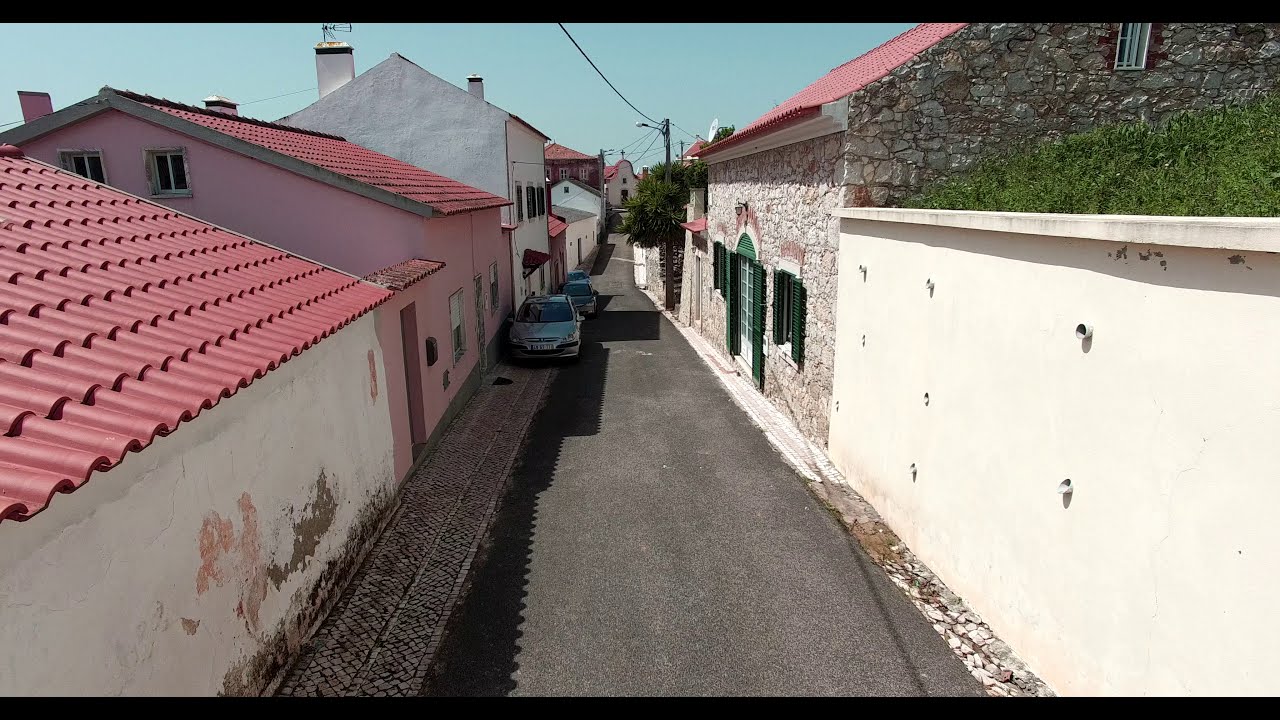This photograph captures a narrow, paved street in a quintessentially European city. Viewed from the center, the street stretches out and slightly disappears towards the horizon under a bright blue, sunny sky. On the left side of the road, there are several small, home-like buildings with white walls and vibrant red-tiled roofs, each varying in height and design. A couple of cars are parked along this side, adding a touch of modernity to the quaint scene. On the right side, the foreground features a white wall with green foliage protruding from the top. Further back, a stone-walled building with a red roof and green-trimmed windows and doors adds to the charming architectural diversity. This building also has a distinct rock decor. Towards the end of the narrow street, one can spot power lines and lighting poles, hinting at the intersection of old-world charm and contemporary amenities in this picturesque European town.